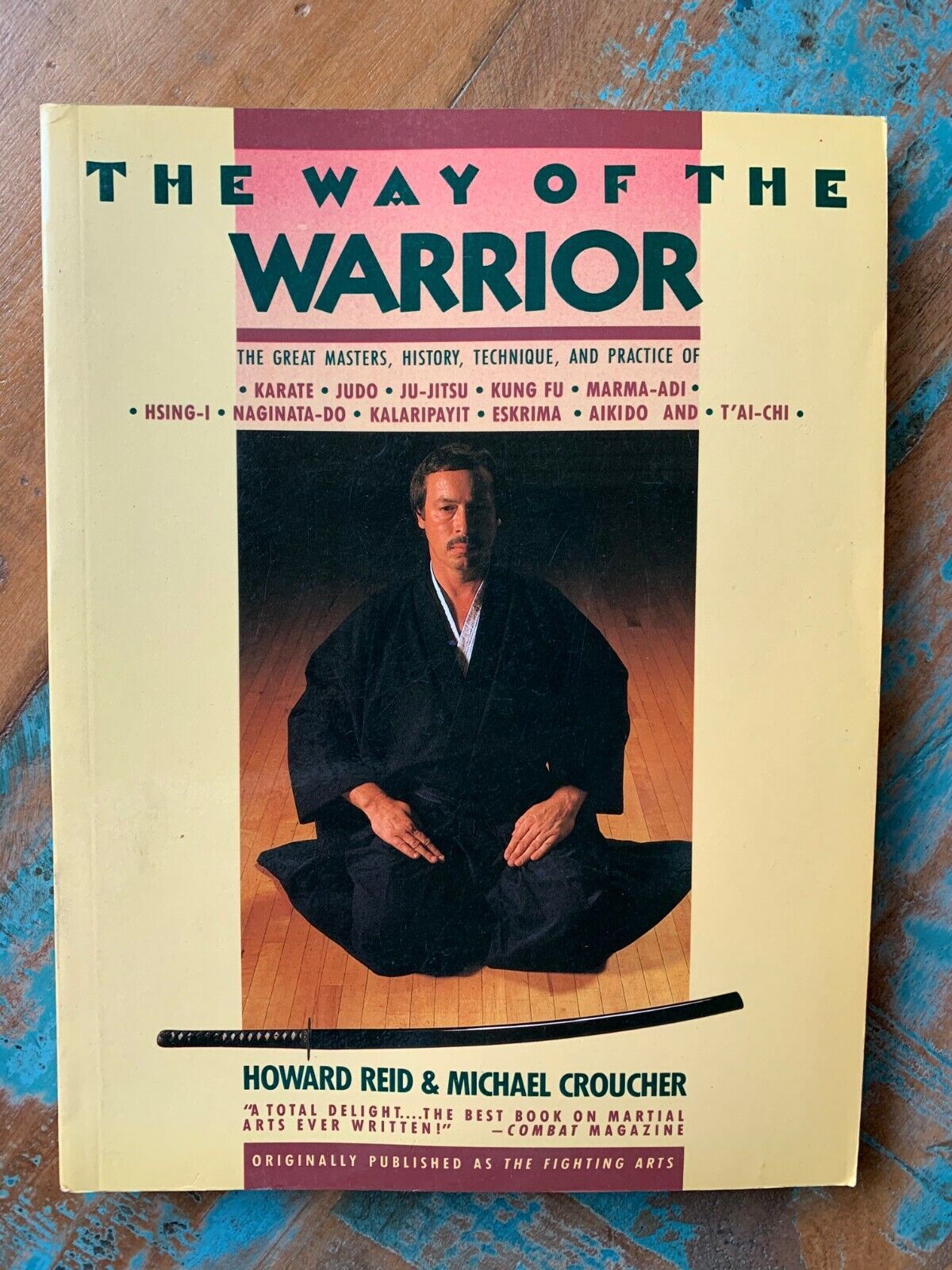The cover of "The Way of the Warrior" prominently features a man meditating on his knees, dressed in a black robe with a white collar peeking underneath, and his hands resting on his legs in a composed manner. In front of him lies a black samurai sword. The book's title, "The Way of the Warrior: The Great Master's History, Technique, and Practice of Karate, Judo, Jujutsu, Kung Fu, Marma Adi, Hsing Ai, Naginata Do, Kalari Payette, Eskrima, Akiro, and Tai Chi," is displayed prominently. Authored by Howard Reed and Michael Croucher, the cover also includes a praise quote from Combat Magazine: "A Total Delight, the Best Book on Martial Arts Ever Written," and notes that it was originally published as "The Fighting Arts." The book is set against a wooden floor background with noticeable blue paint stains, adding texture to the image. The cover itself features a yellow hue with accents of purple, pink, maroon, and navy, enhancing the overall aesthetic of the design.